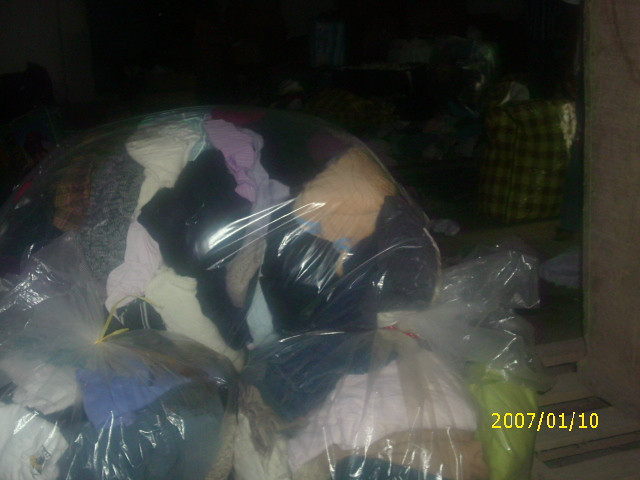This image is an old, poorly lit photograph, possibly a Polaroid, with a timestamp in the bottom right corner reading "2007/01/10." It captures a cluttered scene resembling a hoarder's house, with a dark and chaotic background filled with indistinguishable objects and a plaid item. The focal point is three large, see-through plastic bags piled on top of each other, each stuffed with a colorful assortment of clothes. The clothes inside the bags create a tie-dye effect with colors such as black, purple, white, blue, and orange. The bags are tied with different colored ribbons: one with a red ribbon and another with a yellow one, though the ribbon on the third bag is partly obscured. Due to the low quality and dim lighting, the exact contents of the bags—potentially also containing blankets or towels—are hard to confirm. The overall mood of the image is one of clutter and disarray, suggesting the bags might be intended for donation or disposal.